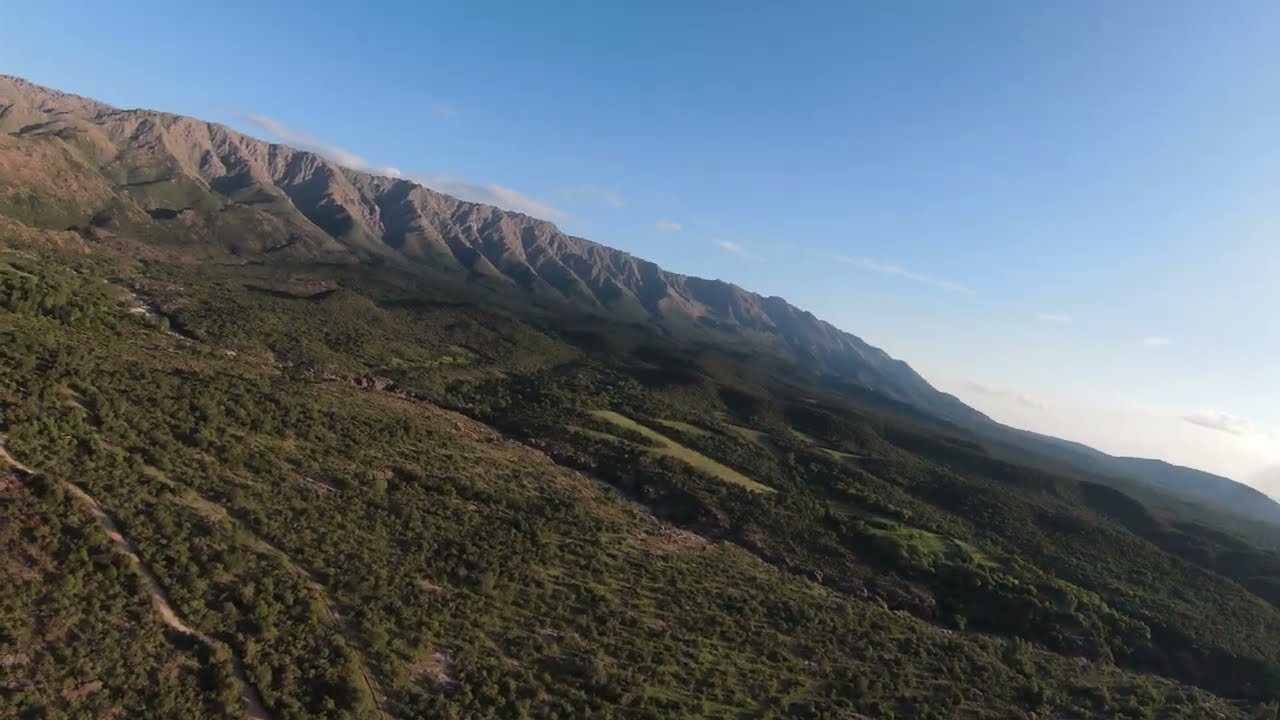This aerial photograph captures a lush, green valley enveloped by various trails and dirt paths that weave through the verdant landscape. As the valley ascends, it transitions into a rocky mountain with a flat top, characterized by its bright brown rock formations. The image is taken at an angle, possibly from a drone or an aircraft, giving a tilted perspective that slopes from the higher left to the lower right. In the background, the blue sky is dotted with small, wispy clouds, and to the right, the sun is setting, casting a serene light over the scene. The image appears slightly hazy, adding to its dreamy quality, with no visible people, animals, or birds in sight, contributing to its untouched and tranquil atmosphere.